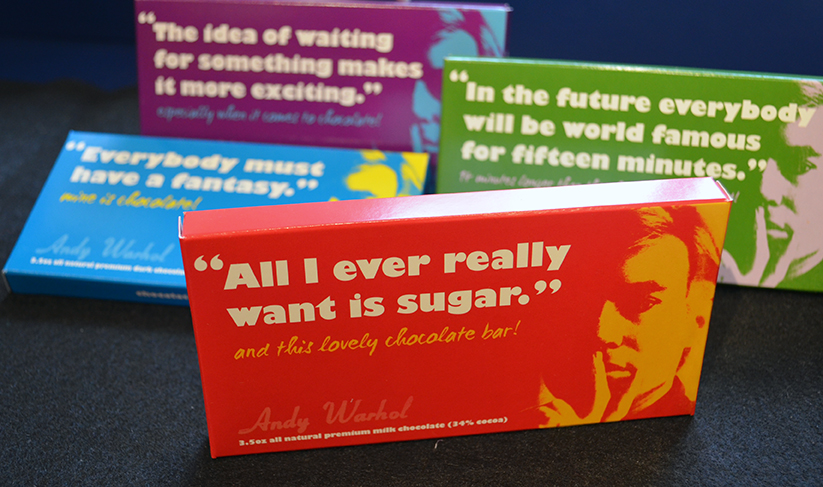The image depicts a collection of chocolate bar packaging, each featuring a different color and quote from Andy Warhol. At the foreground, an orange box prominently displays Warhol's slightly abstract portrait in shades of orange on the right side. Next to his image, in large white text, the quote reads, "All I ever really want is sugar," followed by "and this lovely chocolate bar" in orange brush script below it, with Warhol's name and a line of text underneath. Behind the orange box, other packages of varying colors can be seen. A green box to the right, with a similar design, prominently states, "In the future, everybody will be world famous for 15 minutes." Further back, a blue box lies flat, partially obscured, displaying the quote, "Everybody must have a fantasy," while a purple and blue box at the back reads, "The idea of waiting for something makes it more exciting" in white lettering. Each package, adorned with Warhol's iconic visage, is set against a dark background, giving the scene a vivid contrast. The layout captures the essence of Warhol's art and his reflective quotes, indicating their association with the chocolate bars.